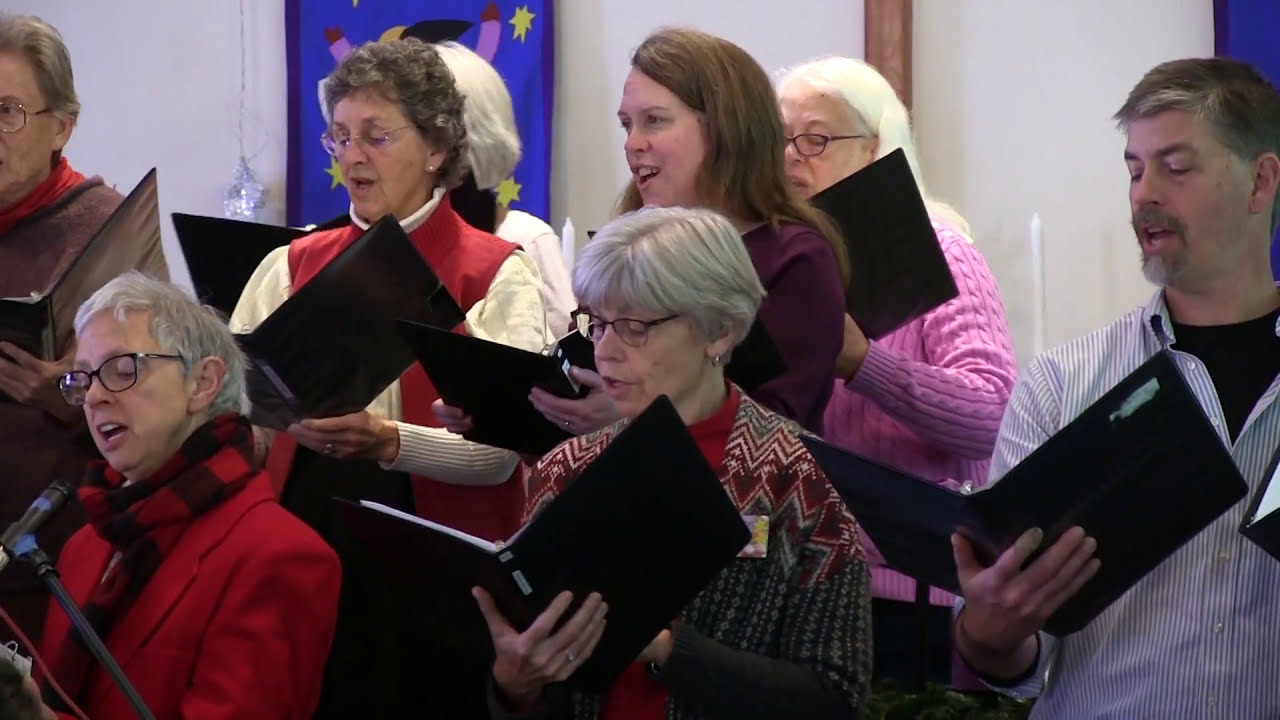The image shows a diverse group of middle-aged to older adults standing in rows, singing together in a choir inside a church. Each choir member holds a black binder in their right hand and appears to be focused on the music, with their mouths partially open in a singing posture. The group includes six women and one man, all dressed in warm attire such as sweaters, coats, and jackets, indicative of cooler temperatures. Notable individuals include a man with a blue shirt and gray goatee, a woman with short gray curly hair wearing golden glasses and a red and white sweater, another woman with long brown hair in a purple sweater, and a woman with a red and brown sweater over a red shirt. The setting has a wooden beam running down the center of the wall and banners reminiscent of a church, including a partially visible blue banner with two yellow stars and a glass star hanging on the white wall in the background.